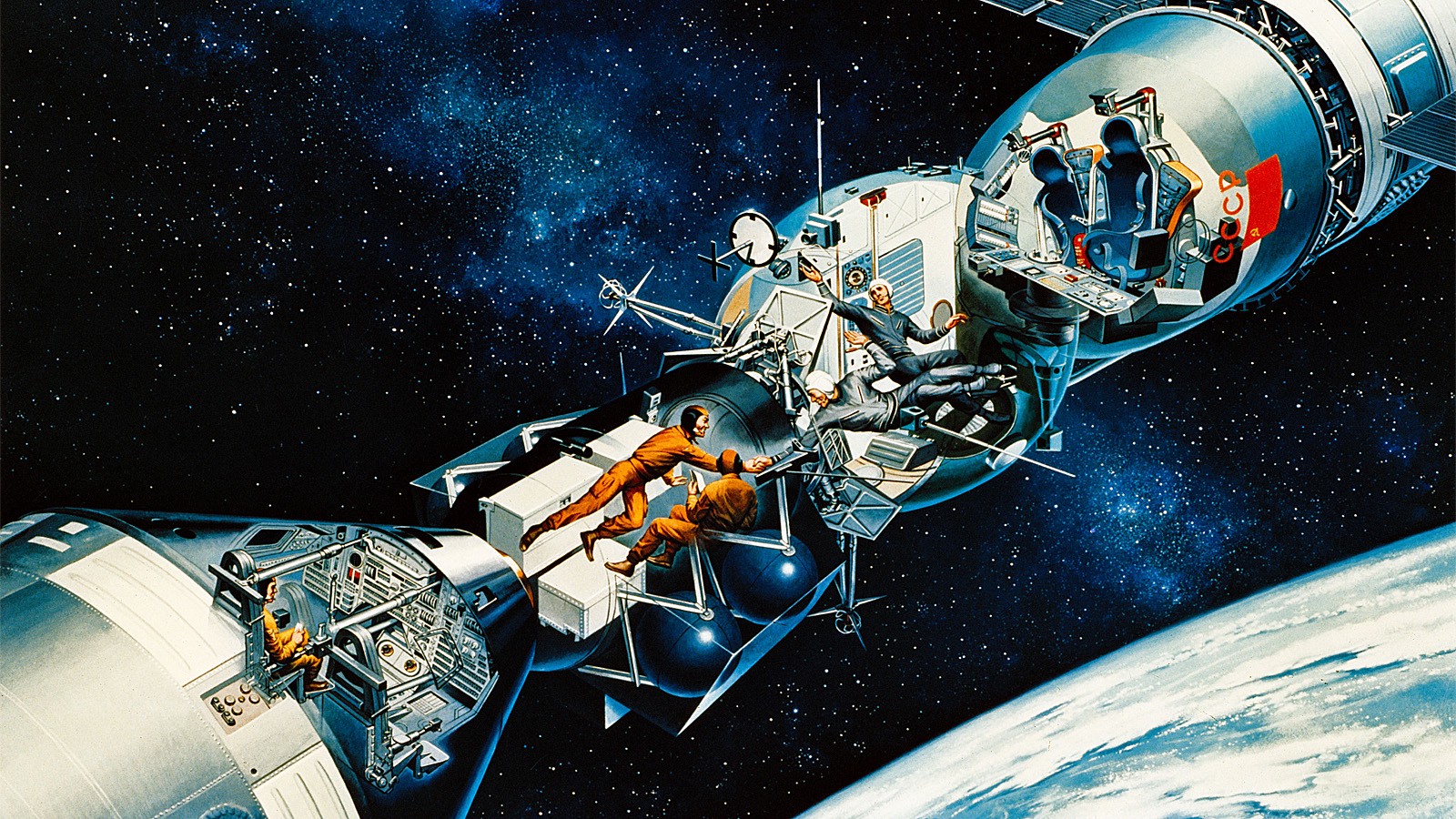The image is a colorful and detailed artistic depiction of a space station set against the blackness of outer space, dotted with numerous bright stars and a prominent lighter band resembling the Milky Way. The space station, stretching diagonally from the lower left corner to the upper right corner, is portrayed without a ceiling, revealing the intricate activities inside. The station bears the red CCCP letters and the old Soviet Union flag. Inside, various astronauts in orange outfits are seen free-floating, engaging in different tasks. One astronaut reaches for another, while another person operates a control panel in the lower left portion. The upper right section shows faint blue shadows that resemble human shapes, though they lack discernible faces. The background also features a blue planet with thick white clouds, potentially Earth, situated in the lower right-hand corner, providing a stark contrast to the dark, star-filled sky.